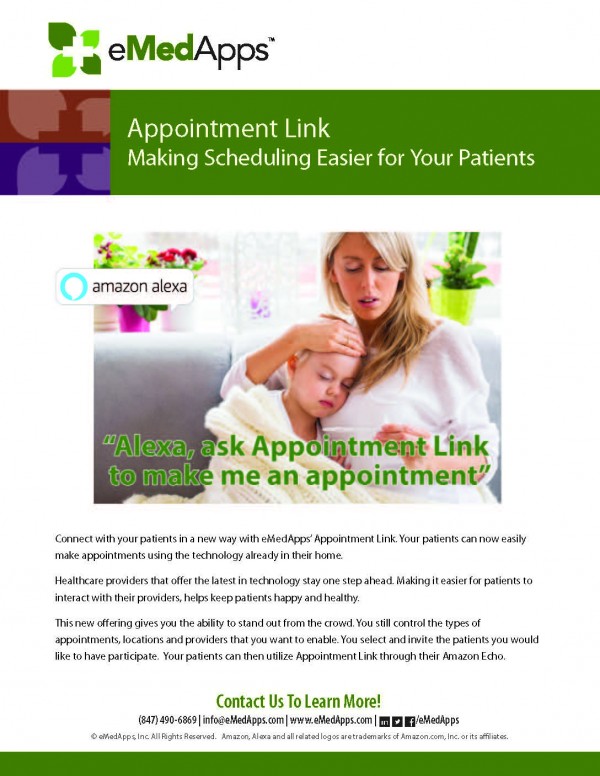This webpage screenshot features a primarily white background at the top, with a logo consisting of four green leaves forming a cross shape in the center. To the right of this logo, the text "eMed Apps" is displayed. Below this is a prominent green rectangle with white text that reads, "Appointment Link: Make scheduling easier for your patients."

Further down, there is a heartwarming photograph of a blonde woman wearing a white robe, holding a blonde boy who is leaning against her chest. The boy, wrapped in a white blanket, is pretending to be sick as the woman gently places her hand on his forehead. 

A green banner across the bottom of the photo includes the text,  "Alexa, ask Appointment Link to make me an appointment."

The section below the photo, in black text, states: "Connect with your patients in a new way with eMed Apps Appointment Link. Your patients can now easily make appointments using the technology already in their home. Health care providers offering the latest in technology stay one step ahead, making it easier for patients to interact with their providers while helping keep patients happy and healthy."